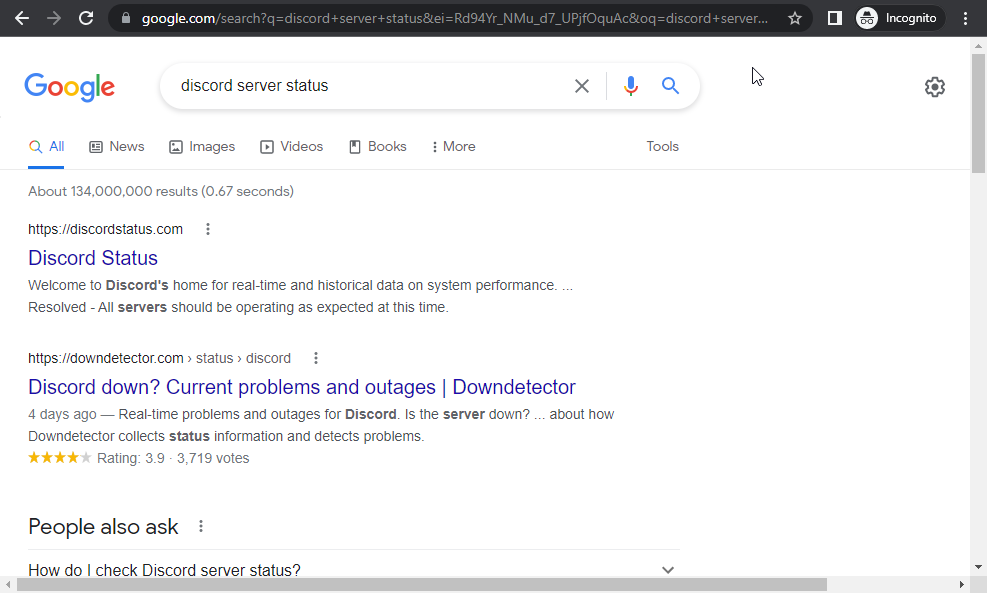The image depicts a Google search results page with the query "Discord server status" entered in the search bar. The text is written in black. The page announces approximately 134 million results retrieved in 0.6 seconds. Two primary search results are prominently displayed.

The first result has the URL "discordstatus.com" with the title "Discord Status" in blue. The associated description reads: "Welcome to Discord's home for real-time and historical data on system performance. Resolved: All servers should be operating as expected at this time."

The second result has the URL "downdetector.com/status/discord" and the title "Discord Down - Current Problems and Outages - Down Detector," dated four days ago. Its description states: "Real-time problems and outages for Discord. Is the server down? Down Detector collects status information and detects problems." This result has a rating of 3.9 stars based on 3,719 votes.

Below these results, there is a "People also ask" section with the query "How do I check Discord server status?" All text on the page is in black, except for the titles, which are in blue. The top left corner of the image features the Google logo in green, blue, yellow, and red.